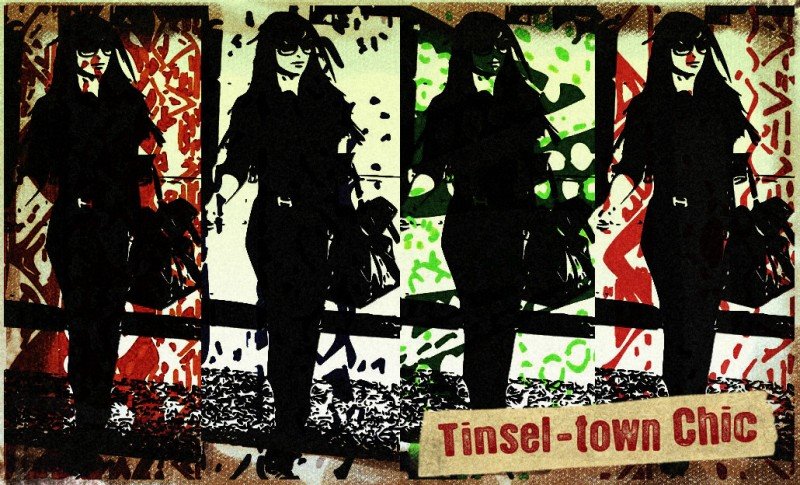The image is a four-panel horizontal collage featuring a sketch of the same woman, likely in her early to mid-twenties, possibly Caucasian or Asian, wearing large sunglasses that obscure her face, a small nose, and pursed lips. Her long, dark hair matches her dark jumpsuit and the large bag she carries in her left hand, while her right hand is free and extended at her side. Each panel presents the woman with varying artistic embellishments: 

- The first (far-left) panel is partially obscured by a dynamic mix of red and black paint.
- The second panel features a predominantly white background with a few scattered leaves and a blackish border at the bottom.
- The third panel sports a green polka dot pattern.
- The fourth (far-right) panel is adorned with red lines and dots.

The entire collage is black and white, with the exception of the colorful overlays in the different panels. At the bottom right corner, a piece of tape appears to be affixed, bearing the red text “Tinseltown Chic.”